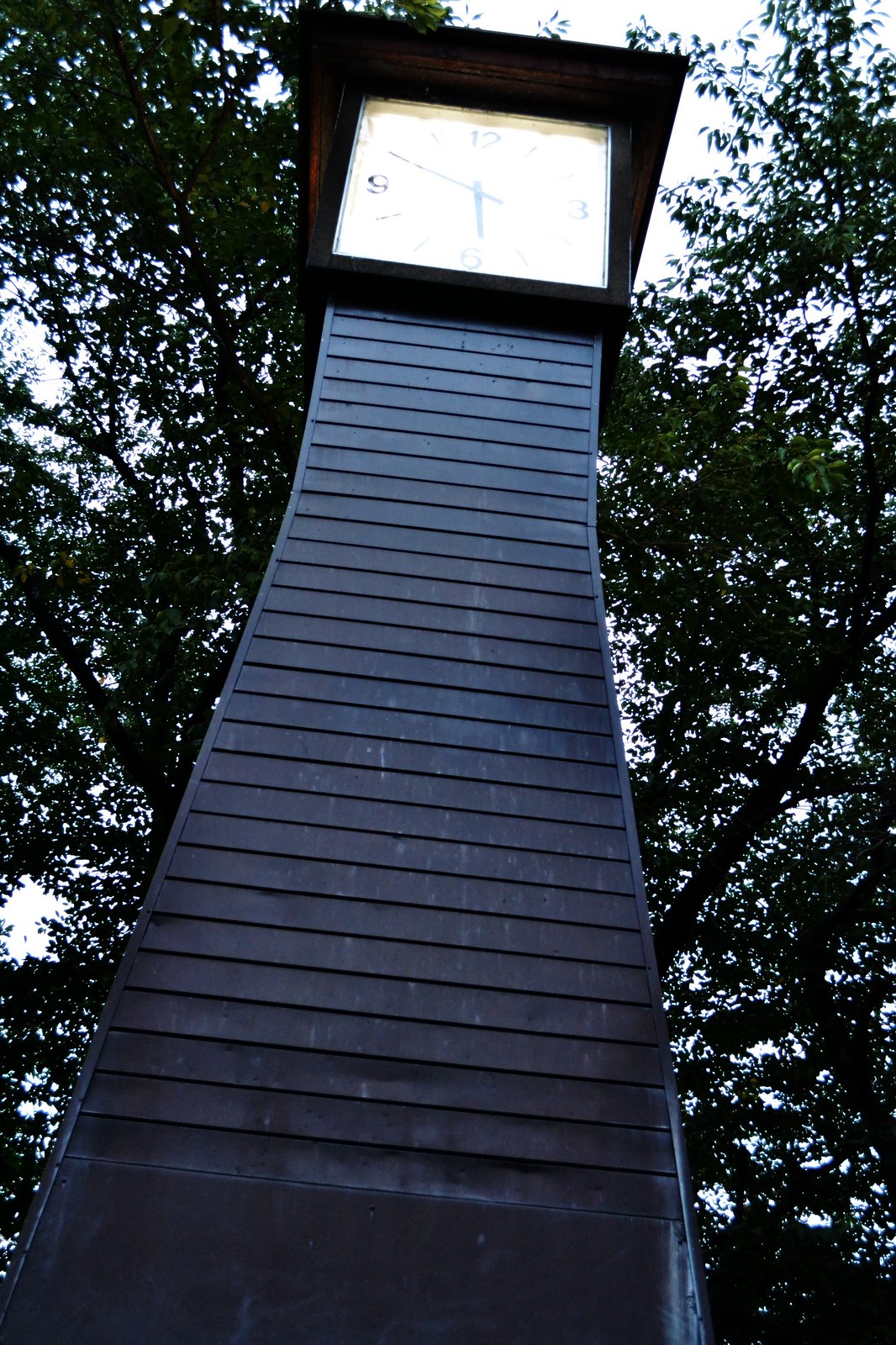A close-up photograph captures a tall, columnar pole that gradually narrows towards the top. Mounted atop the pole is a clock, partially shaded by a protective cover designed to shield it from the elements. The angle of the shot is from below, looking up, revealing an outline of surrounding trees against an illuminated sky. The pole appears to be constructed from wooden planks, adding a rustic texture to the scene. The overall composition emphasizes the interplay of natural and man-made elements, framed by the upward perspective and ambient light.